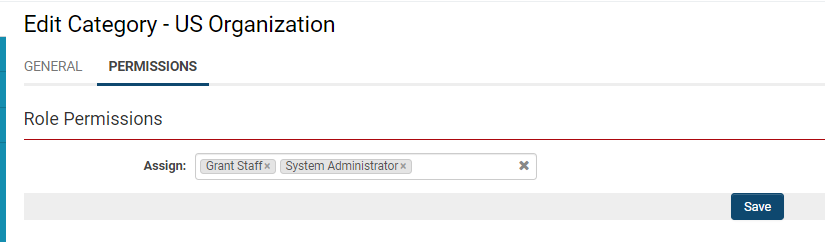The screenshot depicts a section of a website designed for editing categories related to US organizations. The website interface features a clean white background, accented with red lines for subtitles and blue lines for user selections. At the top of the screenshot, the page title "Edit Category - US Organization" is prominently displayed. Directly beneath the title, two tabs are visible: "General" on the left, which is colored grey, and "Permissions," which is highlighted in bold with a blue underline, indicating it has been selected by the user.

Continuing below, there's a heading "Role Permissions" underlined with a thin red line spanning the width of the page. Following this, smaller text labels an "Assign:" section. Accompanying the text is a text box allowing users to type and input options. Entered options appear in grey boxes; currently, "Grant Staff" and "System Administrator" are the existing entries. The bottom right-hand corner features a conspicuous blue "Save" button, providing the user with a clear call to action for saving any changes made on the page.